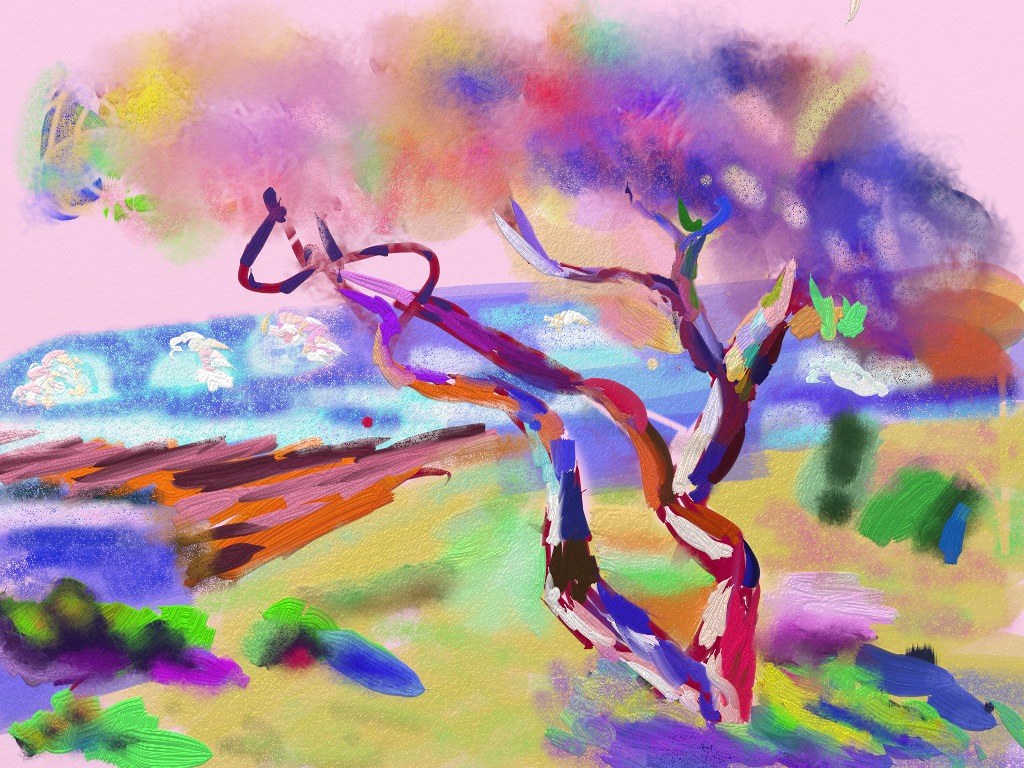This photograph captures a visually striking mixed-media artwork in an abstract style, portraying a vibrant and colorful landscape featuring a lone tree. The sky in the artwork is rendered in a delicate shade of pink, creating a soft yet vivid backdrop. Just above the horizon, a low skyline painted in a calming blue is dotted with fluffy white clouds, adding depth to the scene. Below, a radiant yellow field stretches out, juxtaposed with patches of water illustrated in varying hues of purple and blue, suggesting a reflective surface. The centerpiece of the composition is the tree, its trunk and branches painted in a blend of reds, blues, and purples. The foliage is depicted with expressive blobs of watercolor in an array of purples, yellows, and reds, evoking an image of leaves caught in the light of a setting sun or the bloom of autumn. This piece masterfully combines a spectrum of colors to create a dynamic and emotionally evocative representation of a tree in its landscape.